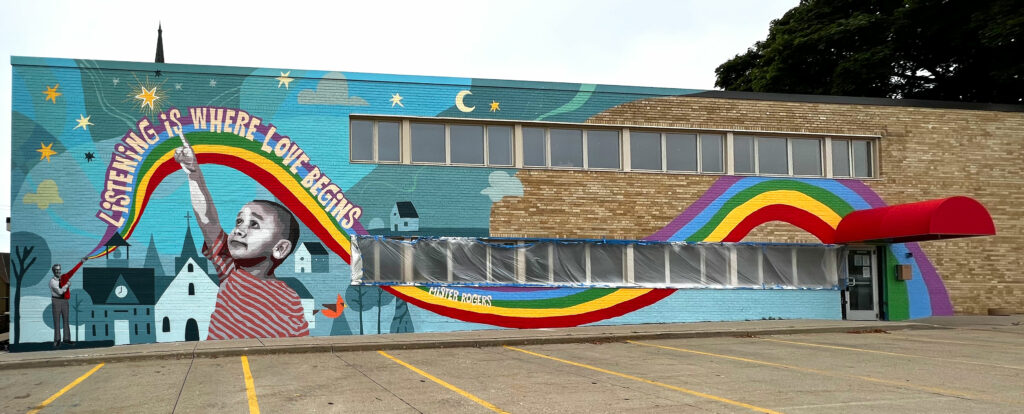The image depicts a large, colorful mural on the brick exterior of a building, possibly a community center or school. The building's facade features varied brick hues of light brown, beige, and dark brown, with more than half of it covered by the vibrant mural. Dominating the scene, the mural's backdrop is primarily a mix of light blue and cyan tones, interspersed with blue screen elements.

Central to the mural is a young African-American boy sporting a red and gray striped shirt, painted in shades of gray. His arm extends upward, with his pointer finger directed at a radiant yellow star emitting beams of light. Behind him stands a man, likely Mr. Rogers, dressed in long sleeves and pants, with frizzy hair. This man holds a red contraption, reminiscent of a bagpipe, from which a swirling rainbow emanates.

The rainbow arcs through the mural, passing behind windows and re-emerging at various points, adorned with text in white letters casting purple shadows that reads, "Listening is where love begins." The rainbow frames scenes of a schoolhouse, farm buildings, and trees. Amidst these elements, Mr. Rogers' name appears in white letters.

A prominent dark green spire, possibly from a church, juts out above the building, enhancing the mural's backdrop under a blue sky. Flanking the scene is a large green tree on the right side. In the foreground, a gray sidewalk and a parking lot marked with yellow lines for spaces emphasize the mural's extent. At the entrance of the building, a long red canopy extends substantially over the silver door, adding a striking architectural element to the composition.